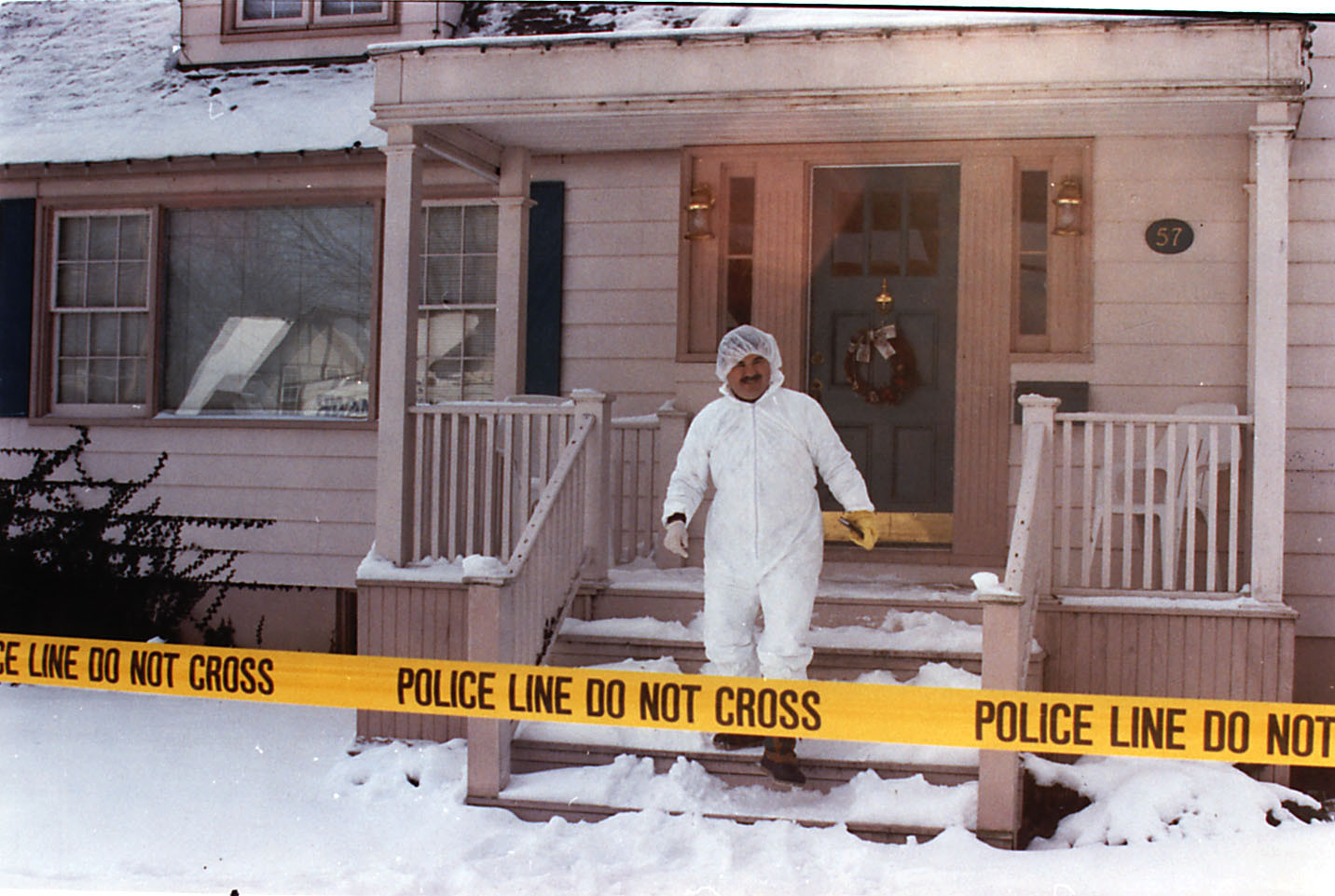In the image, a man dressed in an all-white safety suit with gloves and a plastic hood is captured descending a snow-covered, second step of a house porch. He has a mustache and stands centrally in the frame, directly behind a yellow tape that reads "Police Line, Do Not Cross," suggesting a crime scene. The house, painted a light pink, features a dark green front door with a wreath, and has the number 57 marked to the right of it. The porch and steps are blanketed in snow, continuing onto the ground below and the black-tiled roof above. On the left side of the porch, large windows are visible on both the first and second floors. The setting of the image is outdoors, likely midday, amidst a winter landscape.